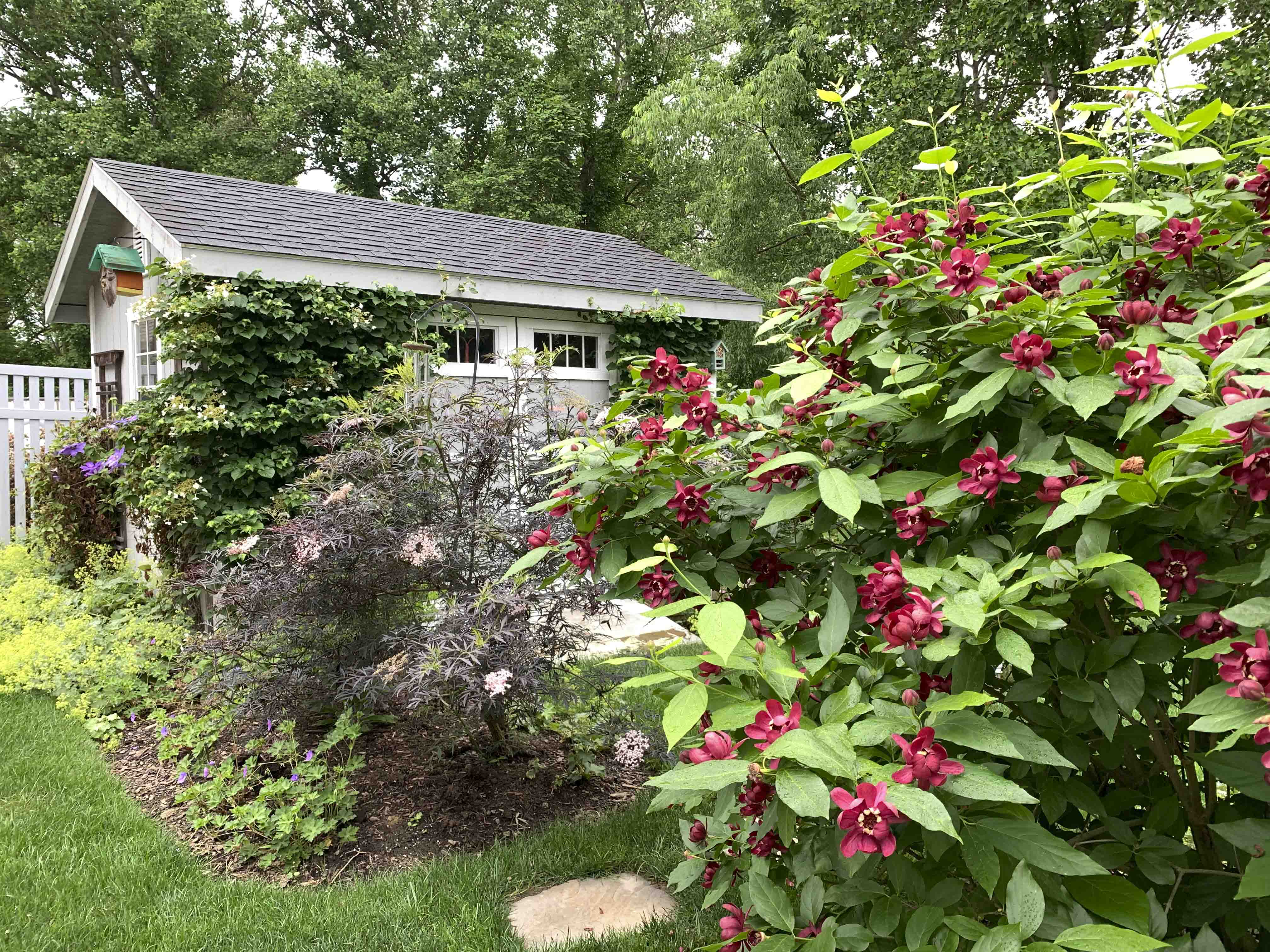This detailed snapshot captures a vibrant backyard garden in the summertime, showcasing an artist's knack for creating a lush, flower-filled haven. In the background, partially obscured by dense greenery and bushes, a small gray garden shed with a slanted roof and white-trimmed windows stands serenely. A birdhouse hangs from one side of the shed, which also features double-sided doors and a stone path leading up to it.

The foreground is dominated by a beautiful, tall flowering shrub with pinkish-red flowers and long, green leaves, creating a striking focal point. Other shrubs and bushes with varying flower colors, including white and purple, add to the rich tapestry of the garden. A large bush with pink flowers and green leaves is prominently positioned on the right, contributing to the diverse array of landscaping plants. Nestled in front of the large red-flowered bush, rock steps are artfully integrated into the ground, enhancing the garden's charming and well-tended appearance. In the background, towering trees frame the scene, creating a serene and secluded environment.